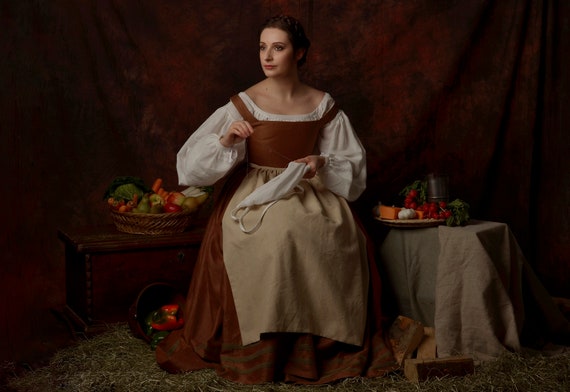The image portrays a light-skinned woman dressed in medieval-style attire, seated against a dark maroon and mottled brown cloth backdrop. She has brown hair pulled back, wears eye makeup and red lipstick, and is adorned in a white puffy-sleeved blouse (chemise) paired with a brown overdress and light brown apron. The setting, which evokes the 15th or 16th century, shows her focusing on sewing a white cloth. Surrounding her is an array of still life elements: on her left side, a tray with garlic, cheese, and possibly radishes and cups; on her right, a basket containing carrots, apples, and possibly a head of cabbage, with additional baskets near her feet that potentially contain peppers. The ground around her features a mix of dark green hues, resembling rushes or woven carpet, contributing to the scene's rustic, historical atmosphere.